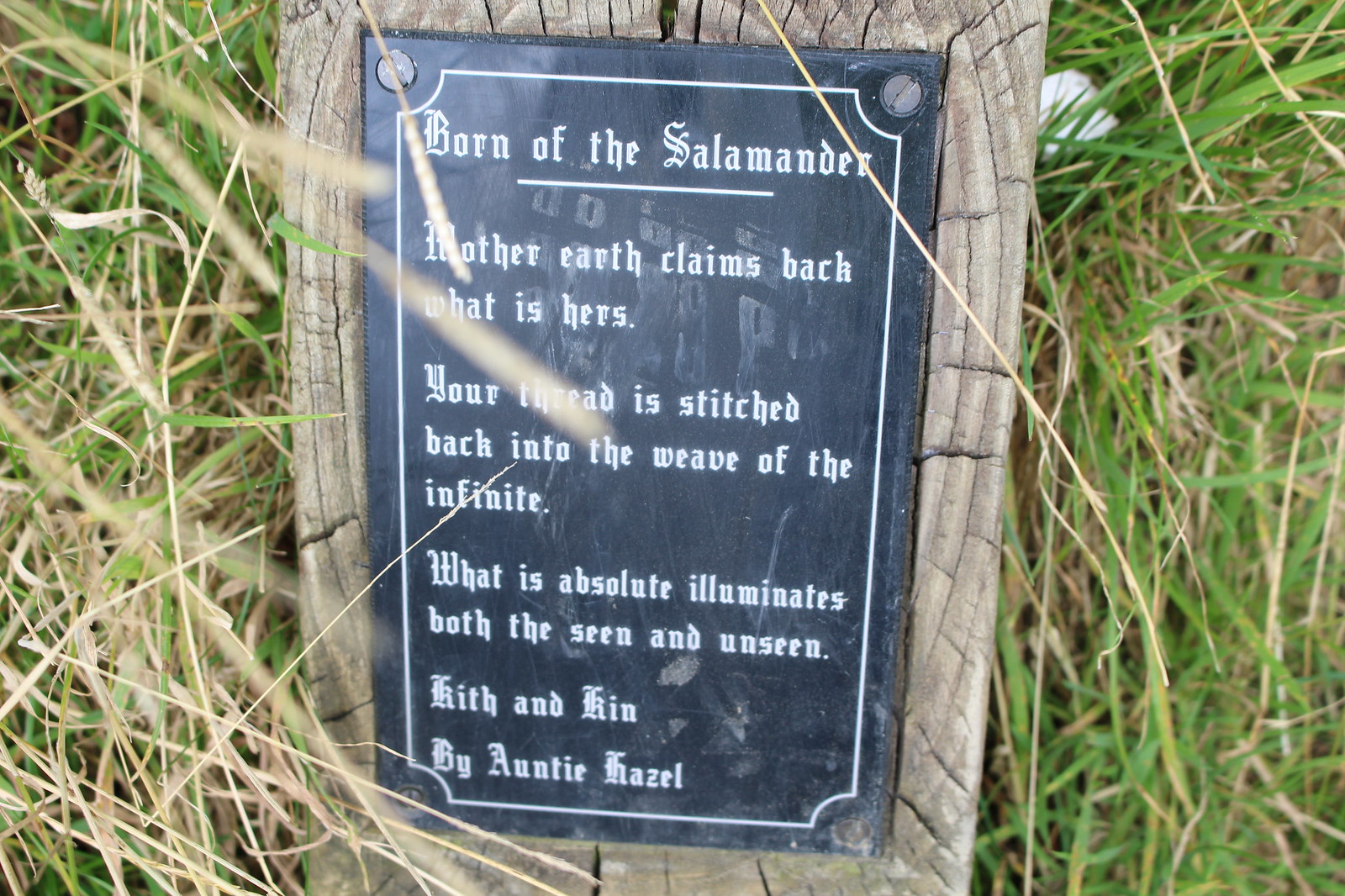The image portrays a weathered sign, possibly serving as a grave marker, affixed to a wooden board. The sign is black with a white border and features white text that reads: "Born of the salamander, that her earth claims back what is hers, your thread stitched back into the weave of the infinite, what is absolute illuminates both the seen and unseen, hit kith and kin by Auntie Hazel." The sign is secured to the wood with bolts in each corner. The wooden board appears to be mounted on what might be a black marble or granite marker. This setup is surrounded by a mix of green, brown, and dead grass, indicating it is situated in a field or cemetery with overgrown vegetation.